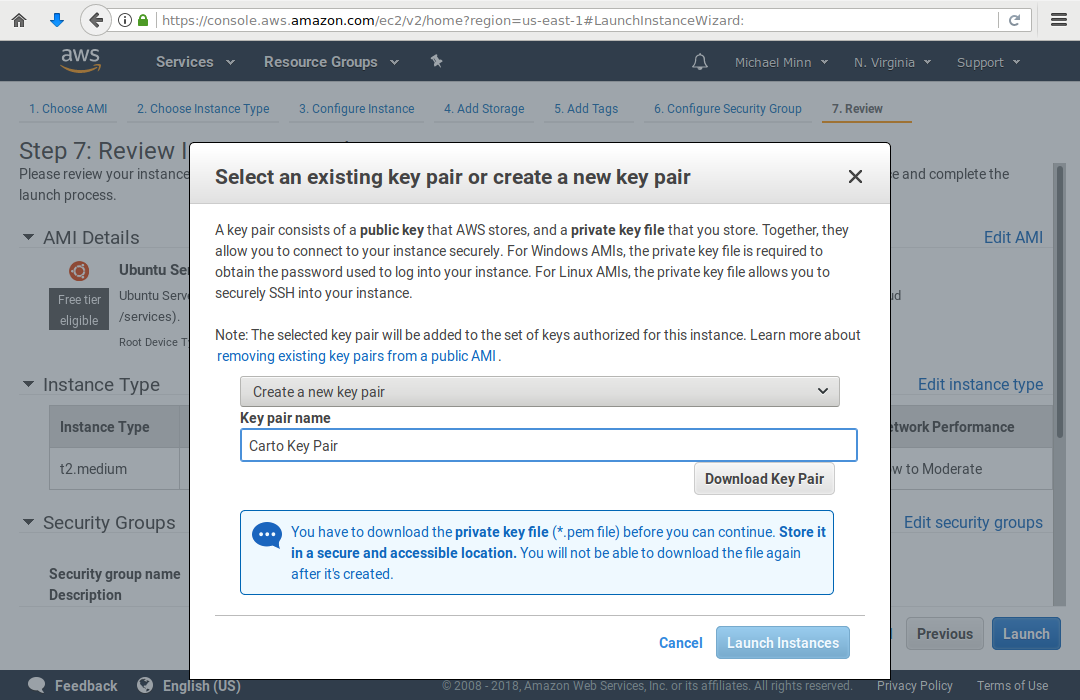Here is a cleaned up and detailed caption for the image described:

---

The image depicts a screenshot of the Amazon Web Services (AWS) Management Console, specifically focusing on the EC2 service. In the background, the familiar AWS logo with the Amazon smile and an upward pointing yellow arrow is seen just above the letter "S." The primary navigation bar at the top includes several drop-down menus labeled "Services," "Resource Groups," a bell icon for notifications, a user profile named "Michael Min" with a drop-down, a region selector set to "North Virginia," and a support drop-down. Above this bar, there is a standard web navigation search bar along with icons for home, a blue down arrow, a left-pointing arrow, an eye symbol encircled, and a lock icon. The URL in the browser bar reads: "https://console.aws.amazon.com/ec2/v2/home?region=us-east-1#launchInstanceWizard."

The page is currently on the "Review" step of the EC2 launch instance wizard, indicated by the highlighted seventh step in black text and a yellow underline. The previous six steps ("Choose AMI," "Choose Instance Type," "Configure Instance," "Add Storage," "Add Tags," and "Configure Security Group") are marked in blue.

A pop-up window is displayed in the foreground. It has a gray header bar with the bold black text, "Select an existing key pair or create a new key pair," and a black X to close the pop-up. Below this, on a white background, is a detailed description explaining that a key pair consists of a public key stored by AWS and a private key stored by the user. It outlines the purpose of the key pair for Windows AMIs (accessing the instance password) and Linux AMIs (secure SSH access). A note mentions that the selected key pair will be authorized for this instance, with a clickable "Learn more" link for additional information about key pairs in public AMIs.

The pop-up includes a drop-down menu currently set to "Create a new key pair." Below this, there is a text box labeled "Key pair name" with the text "Carto" typed inside. A blue "Download Key Pair" button is positioned beneath this text box, followed by a light gray information box with a blue border. This box contains an important message indicating that the user must download the private key file (.pem) before proceeding, emphasizing the need to store it securely as it cannot be downloaded again later. Finally, at the bottom of the pop-up, there are two options: a "Cancel" link and a blue "Launch Instance" button.

---